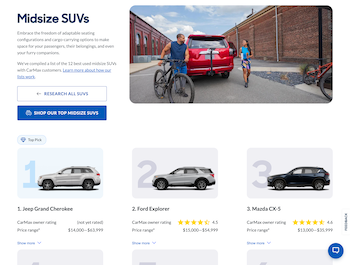This is a screenshot of a CarMax car review and buying webpage dedicated to midsize SUVs. At the top of the screen, the heading "Midsize SUVs" introduces a brief overview of the features and advantages of midsize SUVs. To the right, a prominent banner image showcases a group of people standing in front of a midsize SUV, equipped with bicycles, ready for an adventure—emphasizing the versatile and outdoor-friendly nature of these vehicles. Directly underneath the heading, there's a button labeled "Research All SUVs" followed by another button "Shop Our Midsize SUVs," indicating that this is indeed a car sales website, even though there's no visible logo.

Beneath this section, a series of midsize SUVs are listed, with three specific models currently visible: the Jeep Grand Cherokee, the Ford Explorer, and the Mazda CX-3. Each SUV listing includes a photograph of the vehicle, a CarMax rating, and a price range, helping potential buyers make informed decisions. It's also evident that more SUV options are available if the viewer scrolls down further on the webpage.